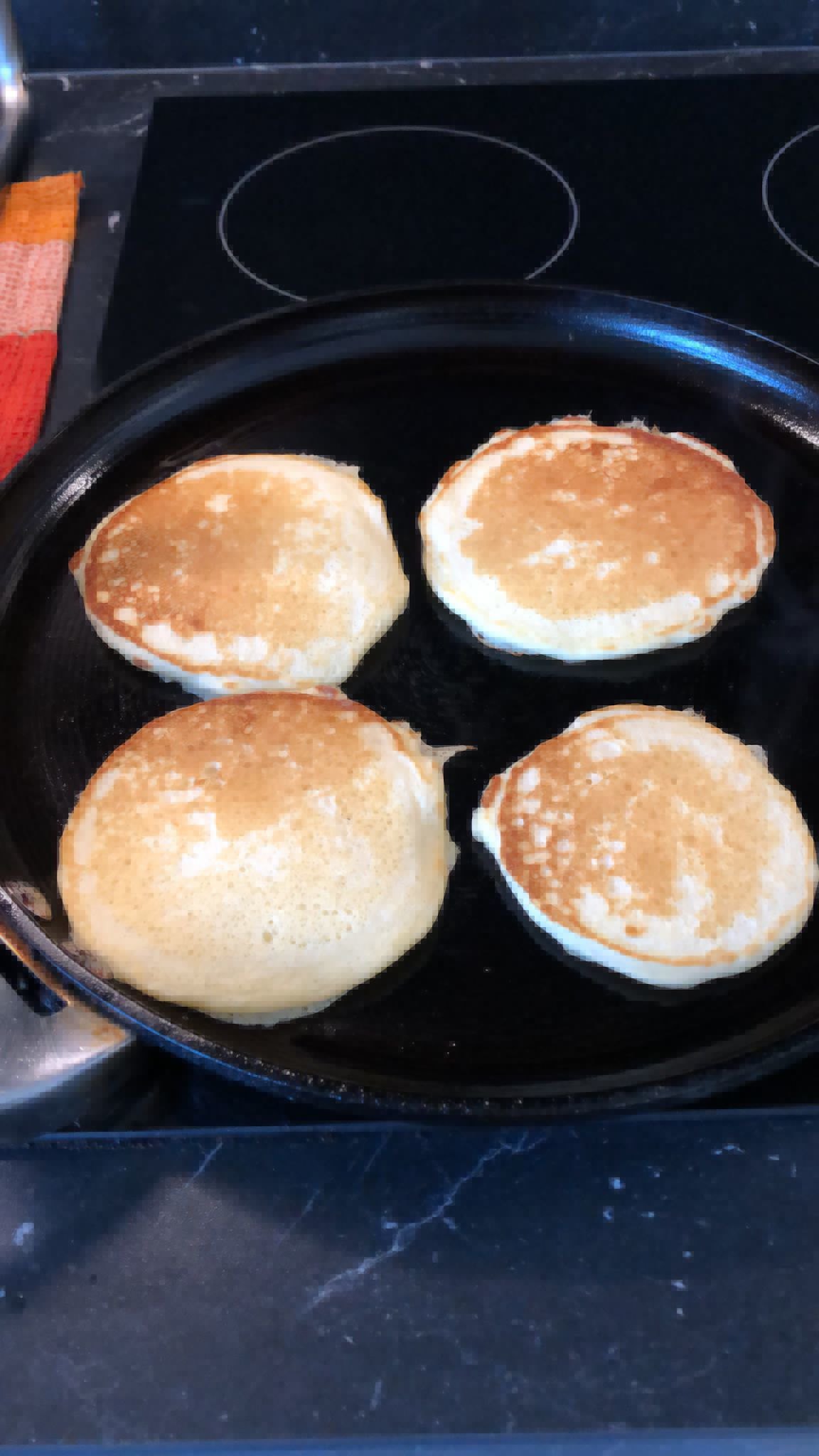This detailed indoor scenic photo showcases a black stovetop with distinctive white circles designating the burners. Positioned centrally on an electric cooktop is a large, black skillet with a faded silver handle angled from the left side. Inside the skillet rest four well-browned pancakes, each varying in size. Notably, the top two pancakes are almost identical, featuring a light brown interior with darker, crispy edges and a lighter bottom. The lower left pancake is the largest, while the lower right one is the smallest. The background comprises a black and white streaked backsplash and countertop. Additionally, an orange, pink, and red cloth is partially visible in the upper left corner, adding a splash of color to the scene.